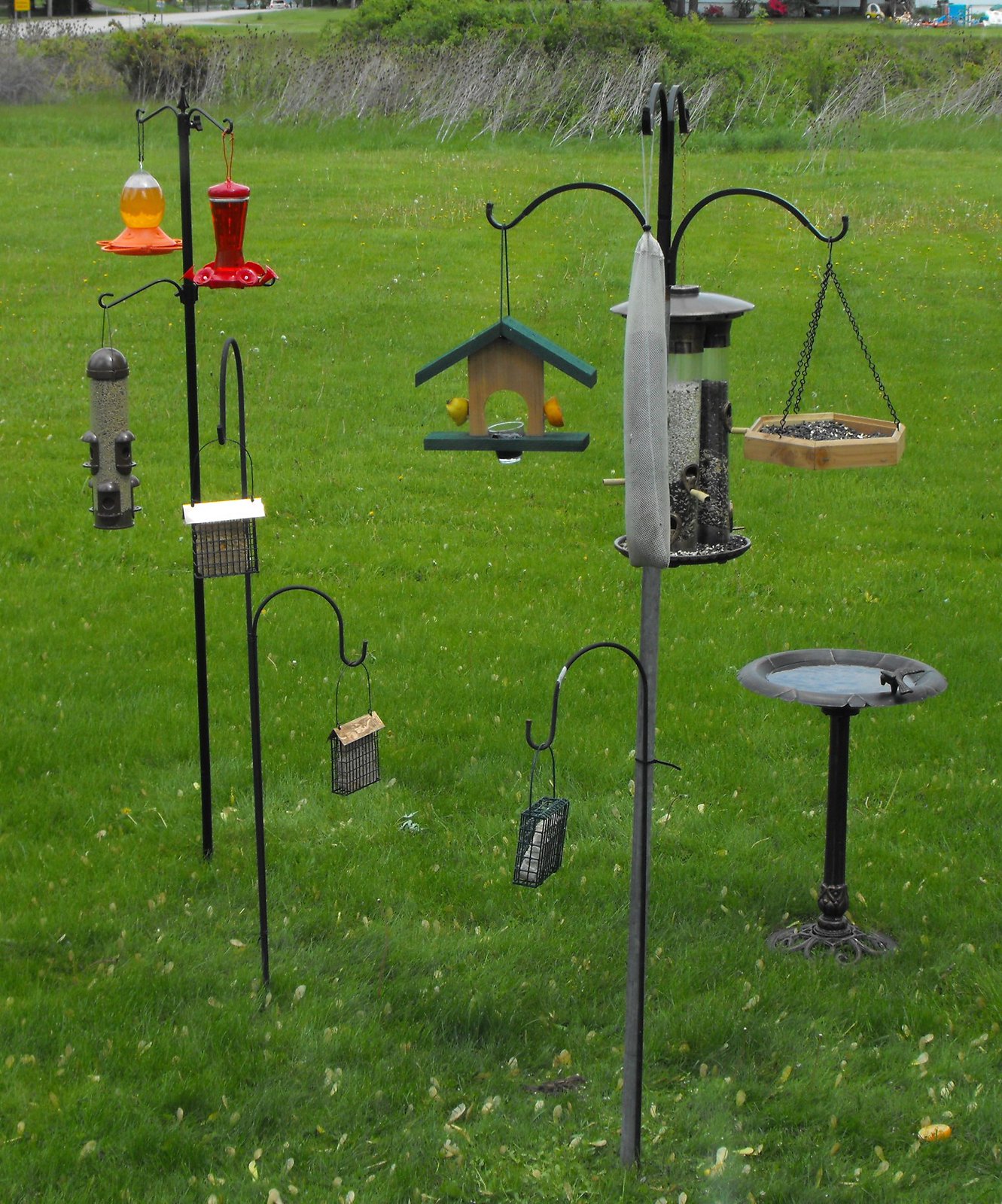This picturesque photograph captures an expansive, lush green backyard that seamlessly transitions into the open countryside. The scene is alive with bursts of yellow flowers and dotted with a variety of bird feeders and birdhouses. On the bottom right, a stone bird bath with a black base provides a serene spot for birds to drink, complemented by a round, classic appearance.

In the foreground, a series of hooks and poles hold a diverse array of bird feeders. One pole, designed like a shepherd's hook, supports several types of feeders: a red hummingbird feeder shaped like a flower with red liquid inside, an orange Oriole feeder, and a standard birdhouse with a green roof and wooden body. A closer look reveals a finch feeder nearly three-quarters full, a suet feeder encased in a metal contraption, and a wooden octagon seed feeder suspended by three chains.

A taller structure supports multiple feeders, including a tri-cylinder feeder for different types of seeds and a finch-specific feeder. There is also another pole featuring three bird feeders at different levels. These feed various bird species, including a long blue feeder and a red container, likely designed for woodpeckers. Additionally, a yellow platform and what appears to be a lamp or light add to the backyard's charm.

In the background, a small pond or lake nestled into a slight gray-stone hill enhances the natural beauty, completing this idyllic birdwatcher's paradise.